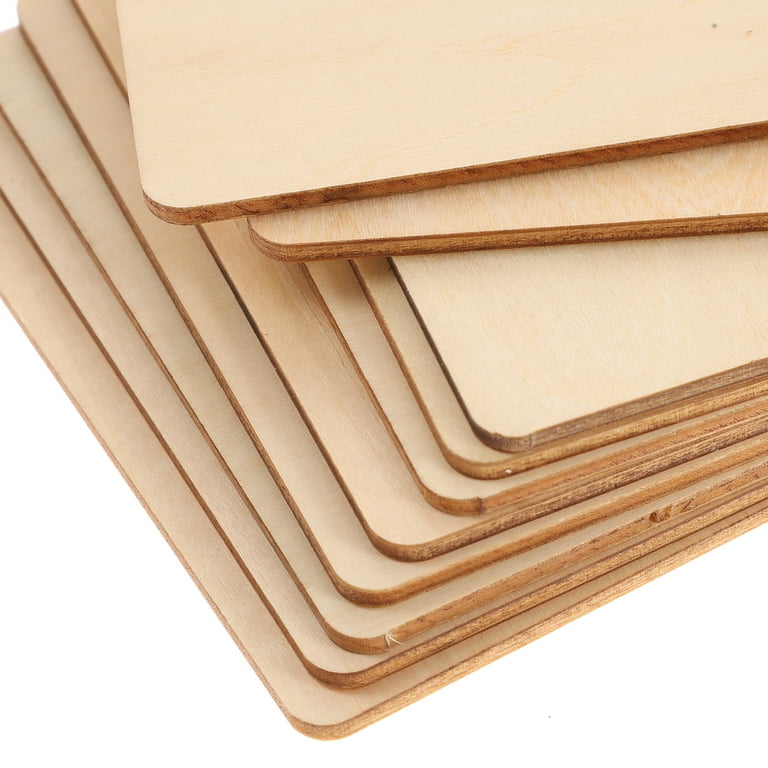A detailed photograph captures a neatly arranged pile of wooden planks or panels set against a plain white background. The planks are square-cut with gently rounded edges, suggesting a balance of both raw and refined craftsmanship. There are approximately ten of these wooden slabs, with the top two slightly disjointed to the top right, creating a subtle shift from the otherwise orderly stack. The rest of the pile ascends diagonally to the right, with each subsequent slab neatly placed on top of the previous one.

Upon closer inspection, the wood exhibits minor imperfections, such as small splinters or 'hangnail' effects, particularly noticeable on the third plank from the bottom. Despite these minor imperfections, the majority of the edges are fairly smooth. The texture of the wood's surface appears well-sanded, contrasting with the slightly rougher edges. This image beautifully highlights the juxtaposition between the natural, rustic qualities of the wood and the careful, methodical arrangement of the planks, evoking a sense of both order and organic beauty.